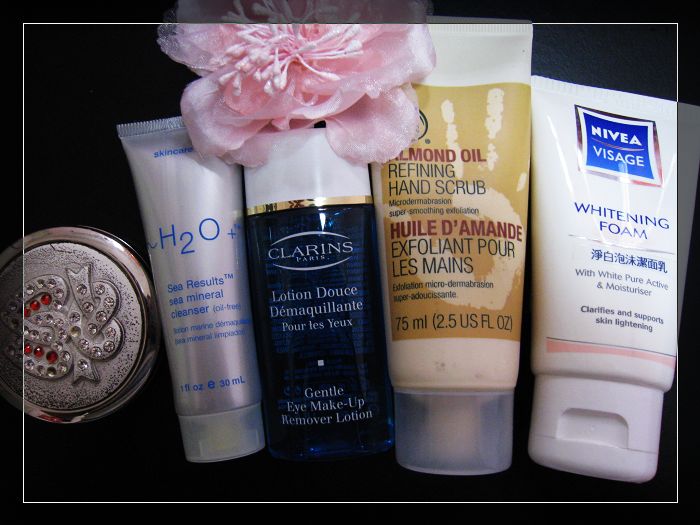In the image, five beauty products are arranged side-by-side against a sleek black background, showcasing an array of skincare and cosmetic items. 

1. The first product is a flat-top circular box, possibly a makeup case. It features a decorative swirl ribbon on the lid, which forms a heart shape adorned with rhinestones, some of which are missing, suggesting frequent use or wear.
  
2. Next, we see a silver tube labeled "H2O Plus Skin Care" featuring the phrase "See Results," cleverly written as "SEA Results." It is a C-Minera Cleanser, incorporating oceanic elements into its skincare formula.

3. The third item is from "Clarins of Paris," named Lotion Douce Démaquillante, which translates to Gentle Eye Makeup Remover Lotion. This product promises to gently cleanse and remove eye makeup efficiently.

4. Following this is the "Almond Oil Refining Hand Scrub," implying a product designed to exfoliate and rejuvenate the skin on your hands with the nourishing benefits of almond oil.

5. The final product in the lineup is "Nivea Visage Whitening Foam," specifically marketed for skin lightening, thereby addressing the needs of consumers seeking a brighter complexion.

Each product stands out against the black backdrop, highlighting their unique packaging and brand identity.